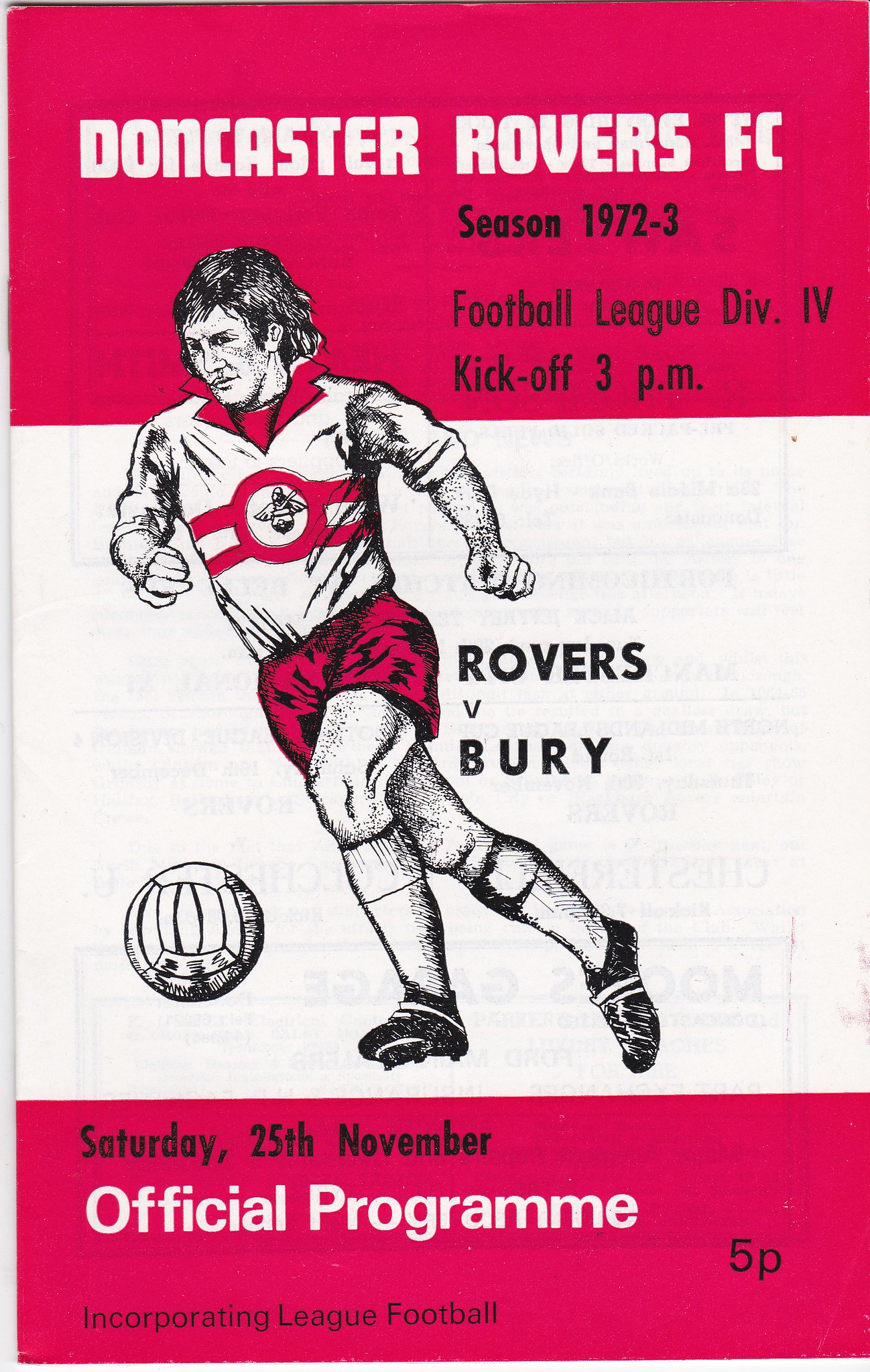The image depicts the front cover of a vintage soccer program from the 1972-1973 season. This vertically-oriented, rectangular program is printed on pink stock with a striking design and dated, muted colors. The top section features a wide, red header with "Doncaster Rovers FC" in quiet uppercase font. Just below, black text reads "Season 1972-73, Football League Division 4, Kickoff 3 p.m." 

The middle, white section prominently displays a black, white, and red line drawing of a footballer running towards the left, ready to kick a soccer ball positioned in front of him. The footballer is dressed in a white and red jersey, red shorts, white socks, and black shoes. Above this illustration, bold black type announces "Rovers vs. Bury."

The bottom section returns to the red color of the header and features several elements in white and black print: the date "Saturday, 25th November," "Official Program," "5p," and the phrase “Incorporating League Football.” The cover likely has some smudges and signs of wear, suggesting it is an older, well-handled program.